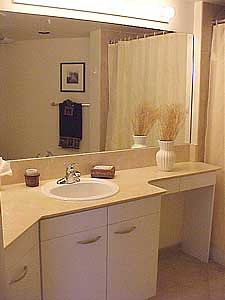This vertical image captures the meticulous details of a modern bathroom interior. Dominating the scene is a large, wide mirror mounted on the wall behind a pristine, white porcelain sink. The sink features a sleek, chrome single-handle faucet. The bathroom's color palette consists of light tannish brown hues, creating a warm and inviting atmosphere.

Resting on the granite or stone countertop are two medium brown containers, symmetrically positioned on either side of the sink. To the right of the sink, in an open space likely designated for a trash can, stands a decorative white vase adorned with a floral design of primarily brown stems and minuscule leaves.

The right edge of the image includes a glimpse of a tan shower curtain, harmonizing with the bathroom's overall color scheme. Reflected in the mirror, dark brown towels hang neatly on a chrome towel bar, underneath a matted photograph in a black frame.

The under-sink cabinet features two doors meeting at the center, each fitted with horizontal chrome handles. To the left, the counter widens slightly, where a box of tissues is placed, adding a practical touch to this elegantly organized space.